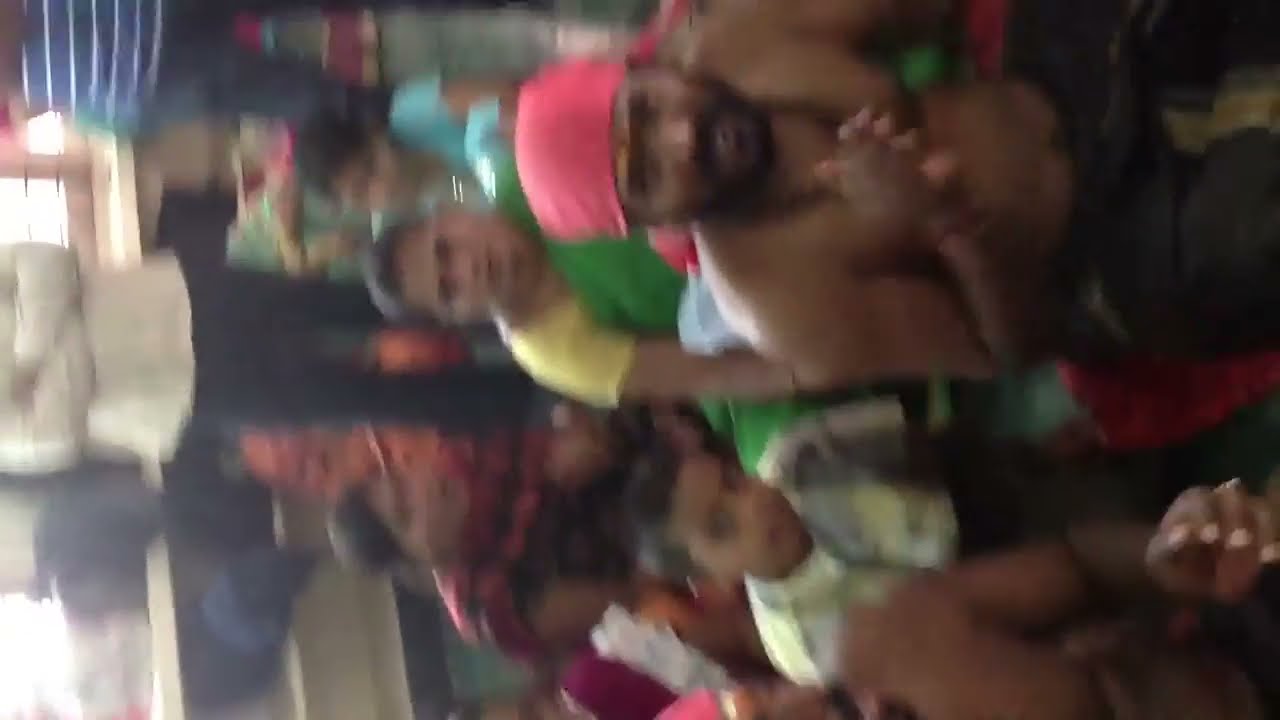The image is a super blurry, sideways photograph of a group of people, with their heads oriented to the left side of the picture and their bodies to the right, suggesting they are seated on tiered steps or bleachers. The central figure is a shirtless man, distinguishable by his red bandana, black pants, and facial hair. To his left is a young child in a short-sleeved shirt of gray and yellow hues. The overall composition captures about eight to ten individuals, mostly men, with varying details such as a younger boy in a white shirt beside the central man, a person in the background standing with arms crossed in a white shirt and black pants, and others in various colored attire, including a yellow shirt with a green overlay and a red and black outfit on a woman. The group appears to be at a busy gathering, possibly a party, where most are looking towards the camera despite the image's poor focus and tilted orientation.